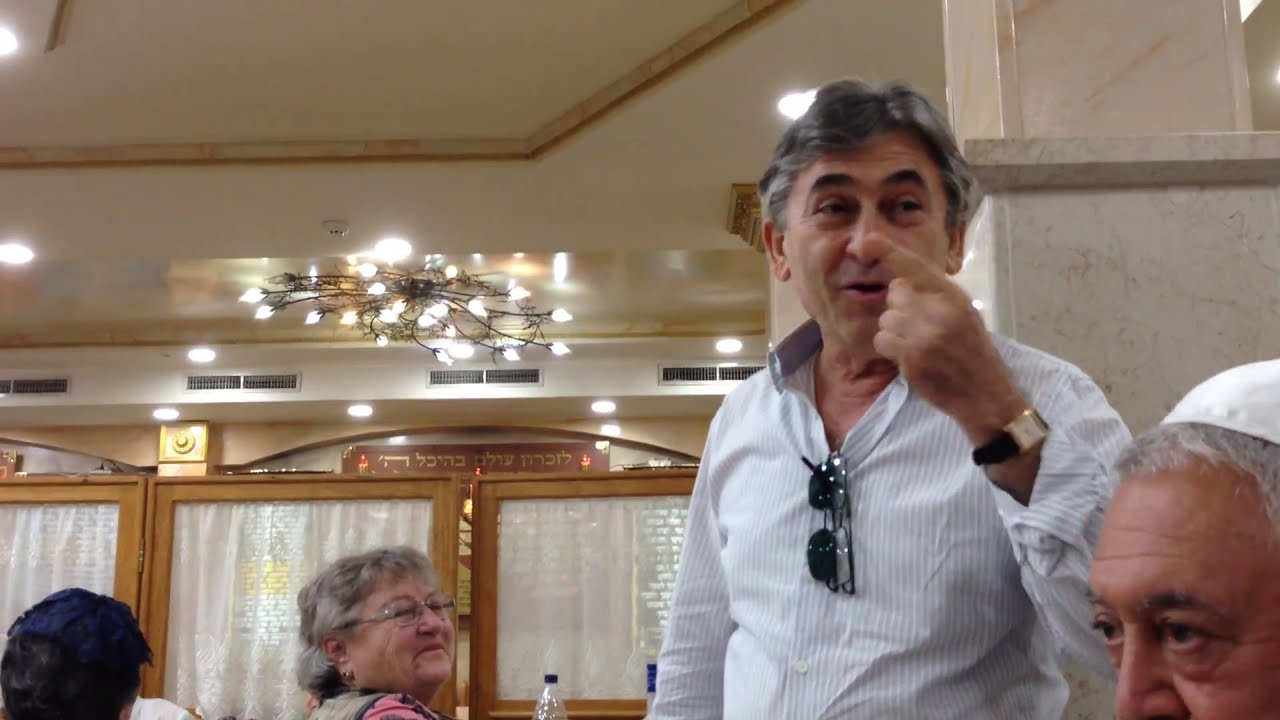The photograph captures an elderly man standing in what appears to be a restaurant or a conference room, characterized by recessed lighting on the ceiling, chandeliers, and marble pillars. The main subject of the image, the elderly man, has wavy, gray hair and well-defined black eyebrows, and he looks to be around 70 years old. He is dressed in a long-sleeved white collared shirt adorned with light gray vertical stripes, from which a pair of black sunglasses is perched. His left wrist bears a black wristwatch with a gold border and white interface, and he's pointing to his right. Behind him, a woman with gray hair, wearing glasses and a gray and red or pink dress, is seated with a bottle of water in front of her. To the right of the main subject, a man wearing a white yarmulke sits with only his eyes, nose, and silver hair visible. The backdrop features white curtains over wooden-framed windows and a door, accentuating what might be a gathering of elder individuals, potentially for a religious ceremony or social event.